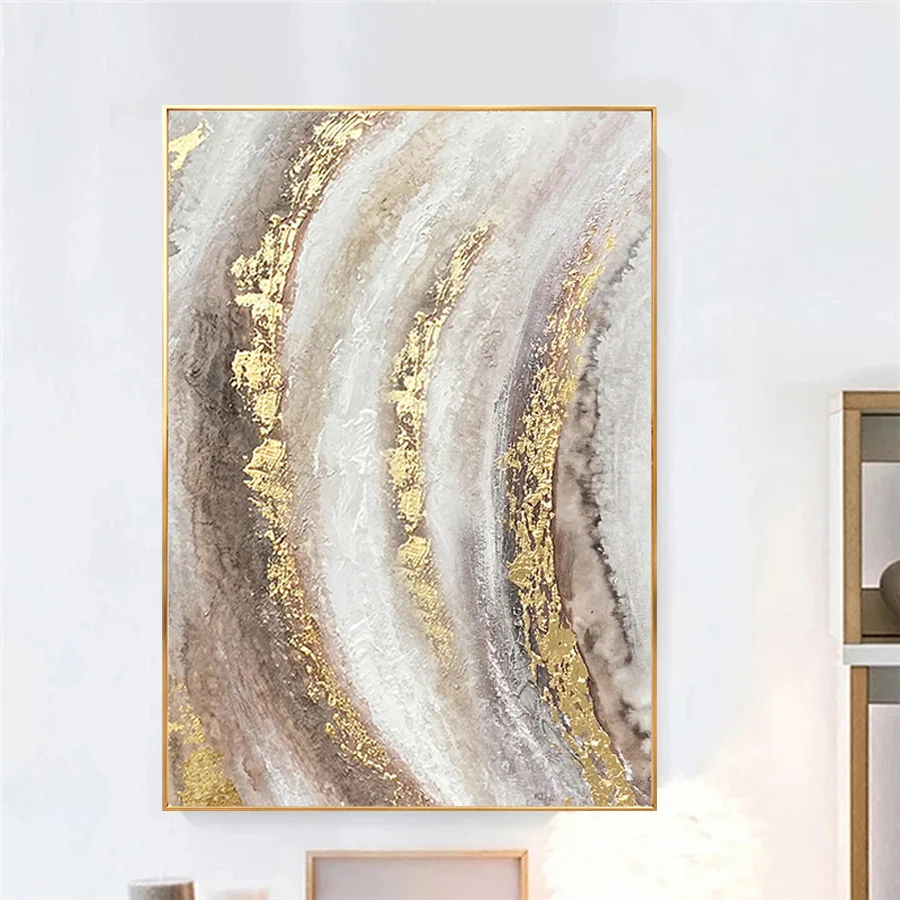The image showcases a vertically oriented, large framed piece of artwork, prominently occupying about 80% of the composition. The artwork is encased in an elegant gold frame, approximately three feet by five feet in size, and is displayed on a white-colored wall. The painting features a textured, abstract design reminiscent of a close-up view of marble or granite. It consists of bold, sweeping brush strokes in shades of brown, gray, and accented with gold. These strokes create curving patterns that start in the middle, arc towards the left, and return to the center near the top, with some hints of pale pink interwoven. Surrounding the primary painting are smaller frames. Below it, there is a brown frame and potentially a lamp or candle. To the right, a wooden shelf with a white laminate edge houses a partially visible round object, possibly a vase. This adds a touch of functional decor to the scene, enhancing the room's aesthetic.